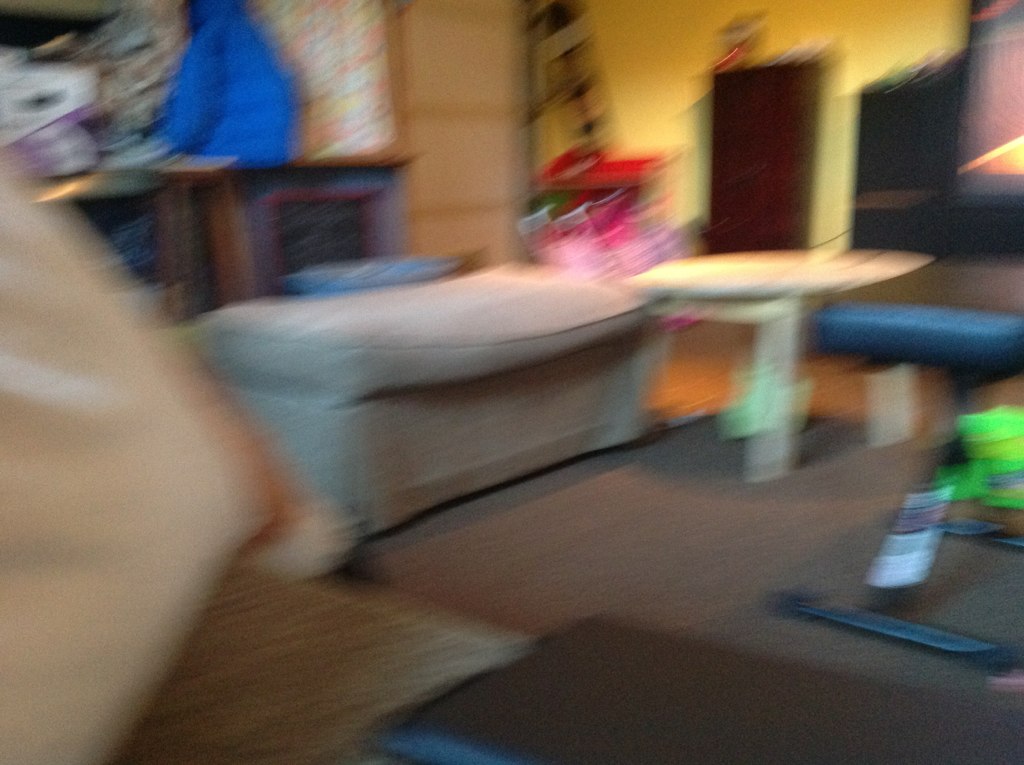This blurry, indistinct photograph captures a room, possibly a living room, lounge, or another shared space such as a waiting area in a building like an apartment, doctor's office, or school. The room features a mix of furnishings and objects in various shades of brown, including a brown carpet and possibly a brown couch with no back, or perhaps a wooden table. Some surfaces appear as rugs or mats layered over a gray carpet. The immediate foreground includes a lighter white table and a tan ottoman.

Towards the right-hand side, there's a black exercise bench adjacent to a lime-green item. There is also mention of what could be a blue exercise bench with tags or papers attached, indicating a less-defined blue object with potential commercial or storage use. The background area suggests more undefined furniture pieces like cabinets or storage bins, with varying colors including green, blue, red, and purple, though the specific items remain indeterminate.

Additionally, there is a blue jacket or some object resembling one hanging on the wall, as well as a wooden door on a yellow wall at the back, potentially marked by an exit sign above it. The photograph is interspersed with lines and visual noise, adding to its overall indistinct and fuzzy quality, making it difficult to clearly identify the exact nature of individual objects in the composition.